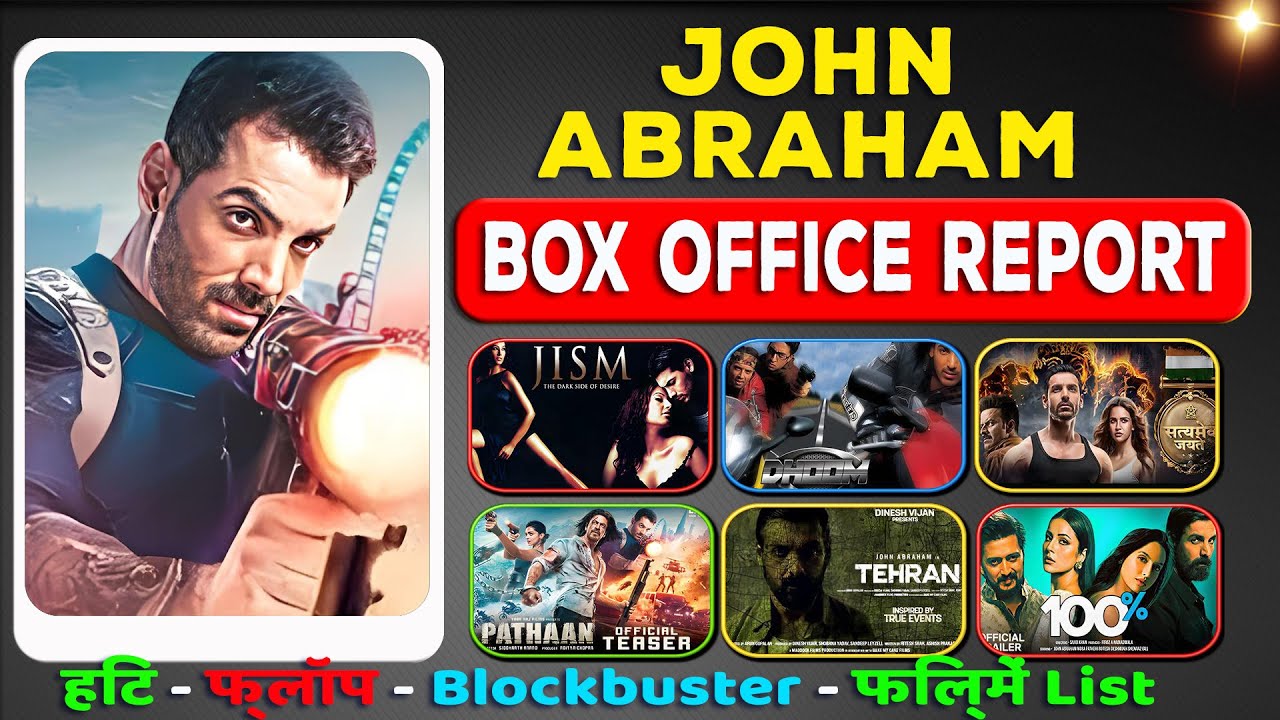The poster depicts an advertisement or box office report for a movie, with intricate detailing. On the left side, there’s an illustration of a man clad in light greenish-blue armor, featuring a dark beard, hair, and eyebrows. He holds a large weapon on his shoulder, emitting a reddish-yellow light. Adjacent to the image, the name "John Abraham" is prominently displayed in yellow, all-capital letters. Beneath this, a red banner with white capital letters reads "Box Office Report." The poster's dark background transitions from black at the top to grey at the bottom, with a spotlight effect illuminating the top right corner. Additionally, the right side showcases six small sections bordered in red, blue, yellow, and green, each displaying different movie titles such as "JISM," "Dhoom," "Path," "Official Teaser," and "Tehran 100%." Text in foreign languages, likely Arabic, appears at the bottom, interspersed with the word "Blockbuster" in light blue at the center.